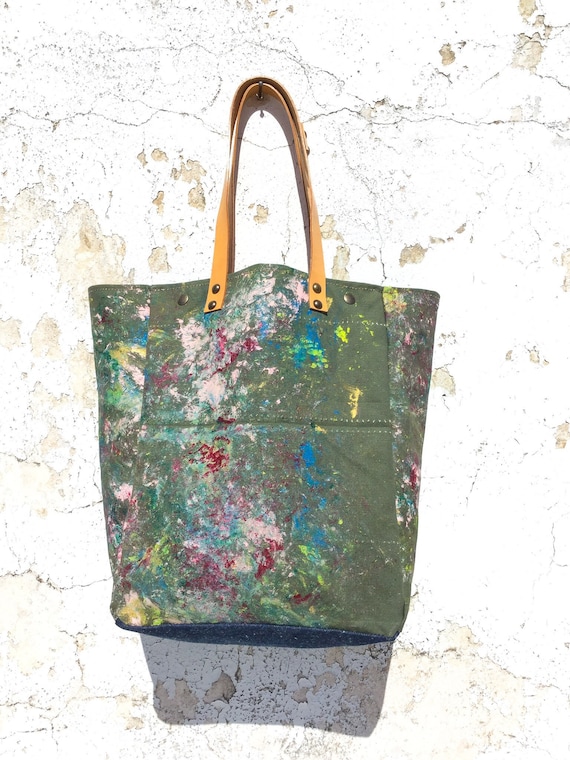The image is a detailed photograph of a tall, tote-style carrying bag with an army gray or olive green canvas background. The bag features two tan leather straps attached to the top with metal studs. It's adorned with vibrant, seemingly random splotches of paint in various colors, including yellow, blue, green, pink, red, and black, giving it an abstract, art-inspired appearance. The paint covers the bag in no particular order, even extending underneath the straps. The photograph captures the bag hanging from a nail on a white, cracked, and peeling wall, which suggests an intentional display setting.